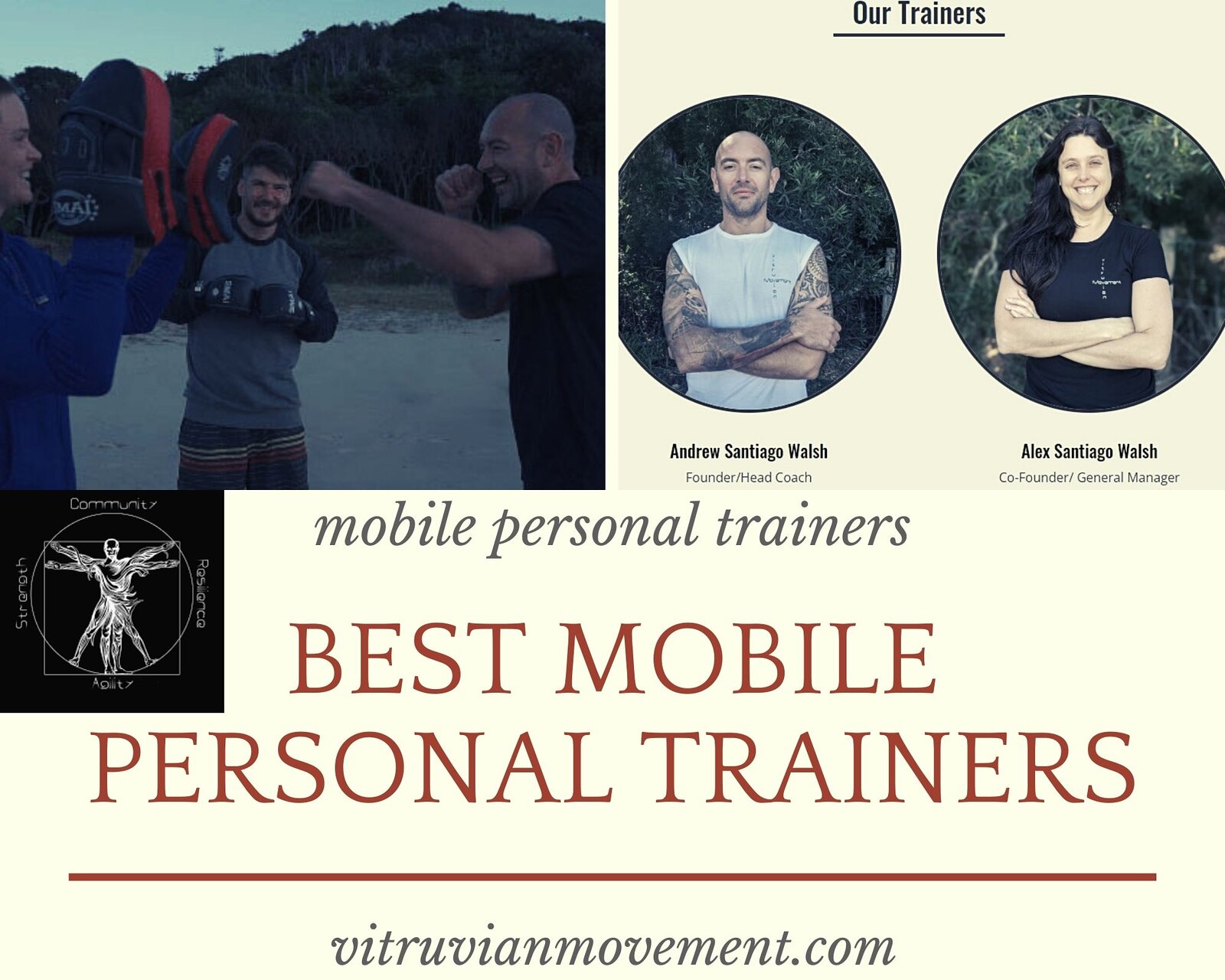The image is a screenshot of a website with a light yellow background, showcasing an advertisement for mobile personal trainers from vitruvianmovement.com. At the bottom of the page, a red line separates the text "Best Mobile Personal Trainers" in red and "Mobile Personal Trainers" in gray. On the top left side, there is a historical drawing by Leonardo da Vinci, displaying two superimposed diagrams of a person with four arms and four legs, symbolizing the ideal human body proportions. Beside this, there's a darker photo featuring three individuals engaged in a boxing training session: a woman with boxing gloves, a man throwing punches at her (both smiling), and another man observing, wearing black gloves. On the top right, there's a heading "Our Trainers" in black, with two circular photographs beneath it. The left photo shows a bald man, Andrew Santigo-Walsh, identified as the founder and head coach, and the right photo displays a woman, Alex Santigo-Walsh, the co-founder and general manager.